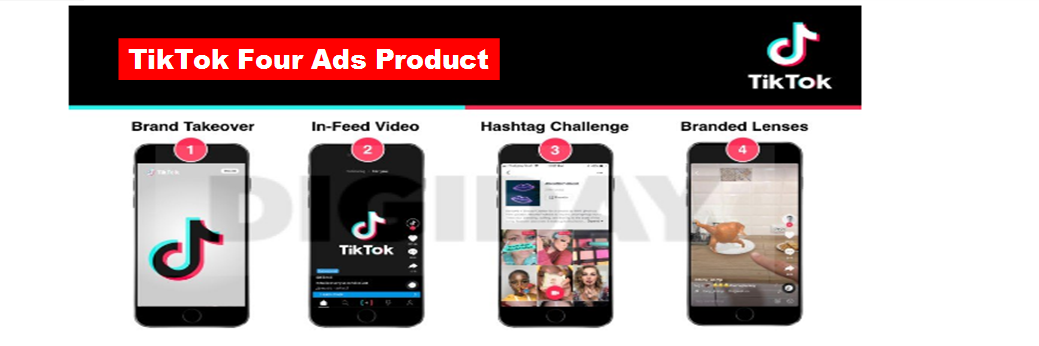This image features a clean, predominantly white background with a prominent black bar at the top, where the TikTok logo is positioned on the right. Displayed on the screen are four smartphone mock-ups, each highlighting different TikTok advertising products. The first smartphone displays a "Brand Takeover" ad, the second showcases an "In-Feed Video," the third highlights a "Hashtag Challenge," and the fourth features "Branded Lenses." The color scheme incorporates black, red, white, and blue elements, creating a cohesive and visually appealing layout. The text across the top reads "TikTok for Ads Product," indicating the range of advertising options available on the platform.